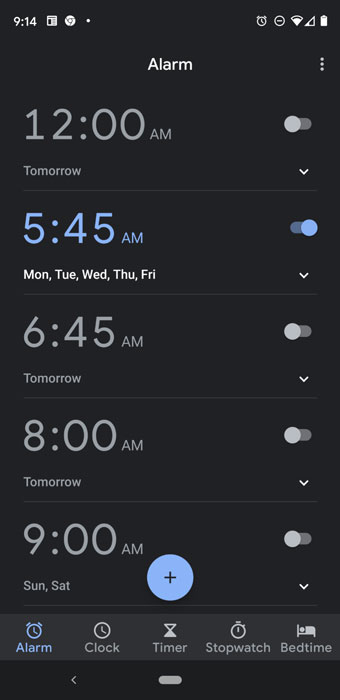The image is a vertical screenshot of an alarm screen on a cell phone. The current time displayed at the top is 9:14. At the upper left-hand corner, there are three small icons, and at the upper right-hand corner, there are five small icons. Centrally positioned is the word "Alarm," accompanied by three vertical dots on its right side. 

The main section displays five alarms:
1. **12:00 AM** - This alarm is turned off and is set for tomorrow.
2. **5:45 AM** - This alarm is turned on, highlighted in blue, and scheduled for Monday through Friday.
3. **6:45 AM** - This alarm is set for tomorrow but is currently turned off.
4. **8:00 AM** - This alarm is also turned off.
5. **9:00 AM** - This alarm is turned off and set for Sunday and Saturday.

Each alarm entry has a slider bar on the right side to toggle it on or off, and a white arrow for accessing drop-down options.

At the bottom of the image is a dark gray banner featuring five icons labeled "Alarm," "Clock," "Timer," "Stopwatch," and "Bedtime." Both the "Alarm" icon and the word "Alarm" are highlighted in blue, indicating the current active section.